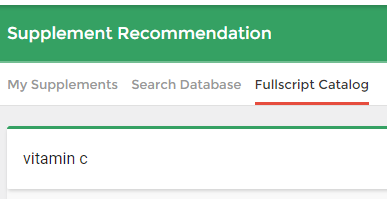A screenshot likely captured from an application or website interface, showcasing a section dedicated to supplement recommendations. At the top, there's a green horizontal bar with the white text "Supplement Recommendations." Directly beneath this, there's a white horizontal menu featuring three navigational options: "My Supplement Search," "Database," and "Full Script Catalog." Following this menu is another white horizontal bar displaying the text "Vitamin C." The screen capture is cut off just below the word "Vitamin C," leaving the lower content obscured.